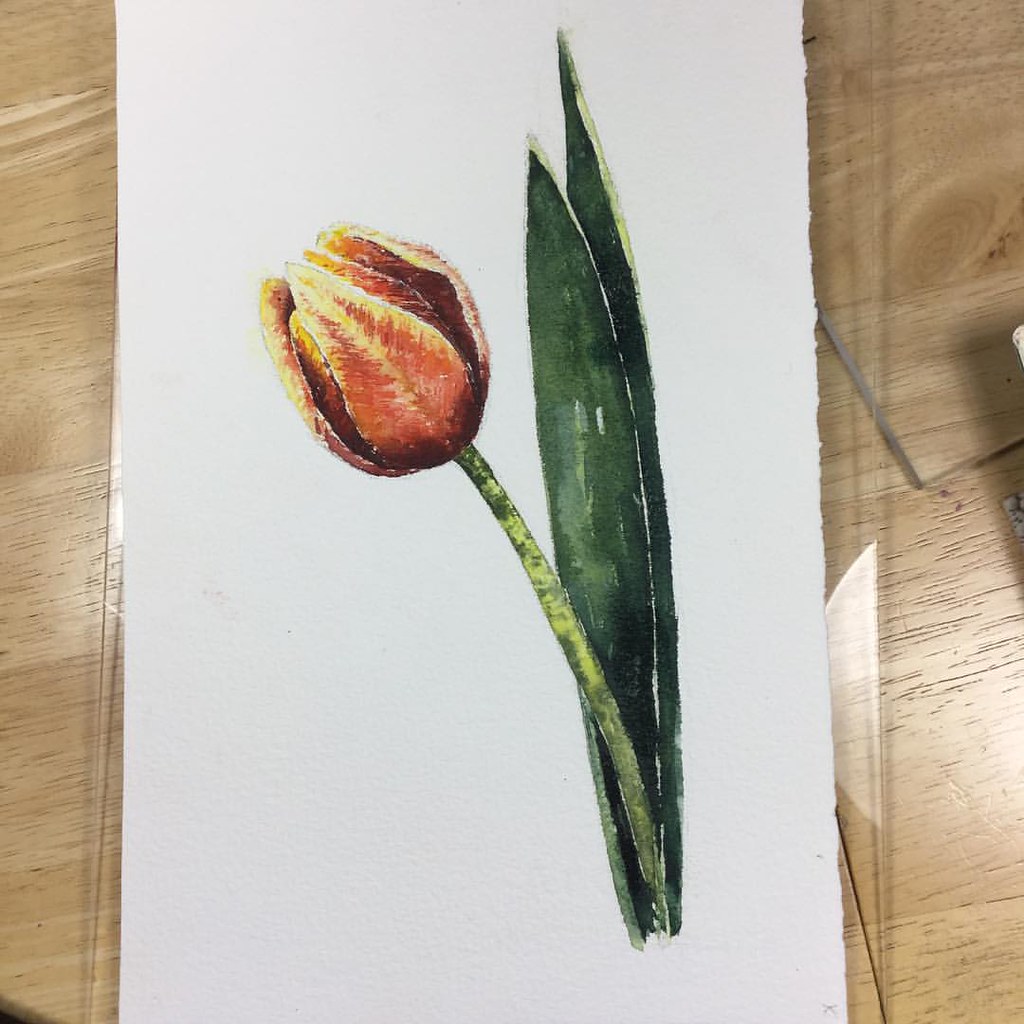This image shows a detailed artwork of a tulip on a white piece of paper, which rests on a light-colored wooden tabletop. The paper appears to be torn on the right side. The tulip features a long, thick stem painted in shades of green watercolors, with hints of light and dark green for depth. Two large, pointy leaves flank the stem, also rendered in dark green with lighter green tips and subtle shadowing. The flower itself is illustrated with colored pencils in vibrant hues of yellows, oranges, and deep rust colors, suggesting a tulip that is on the verge of blooming. The petals appear closed in on themselves, with additional yellow accents visible at the edges, enhancing the realism. The crimson and burgundy tones blend seamlessly, with additional hints of yellow specks reminiscent of natural tulip petals. The overall composition creates a striking contrast against the textured wood grain background of the tabletop.